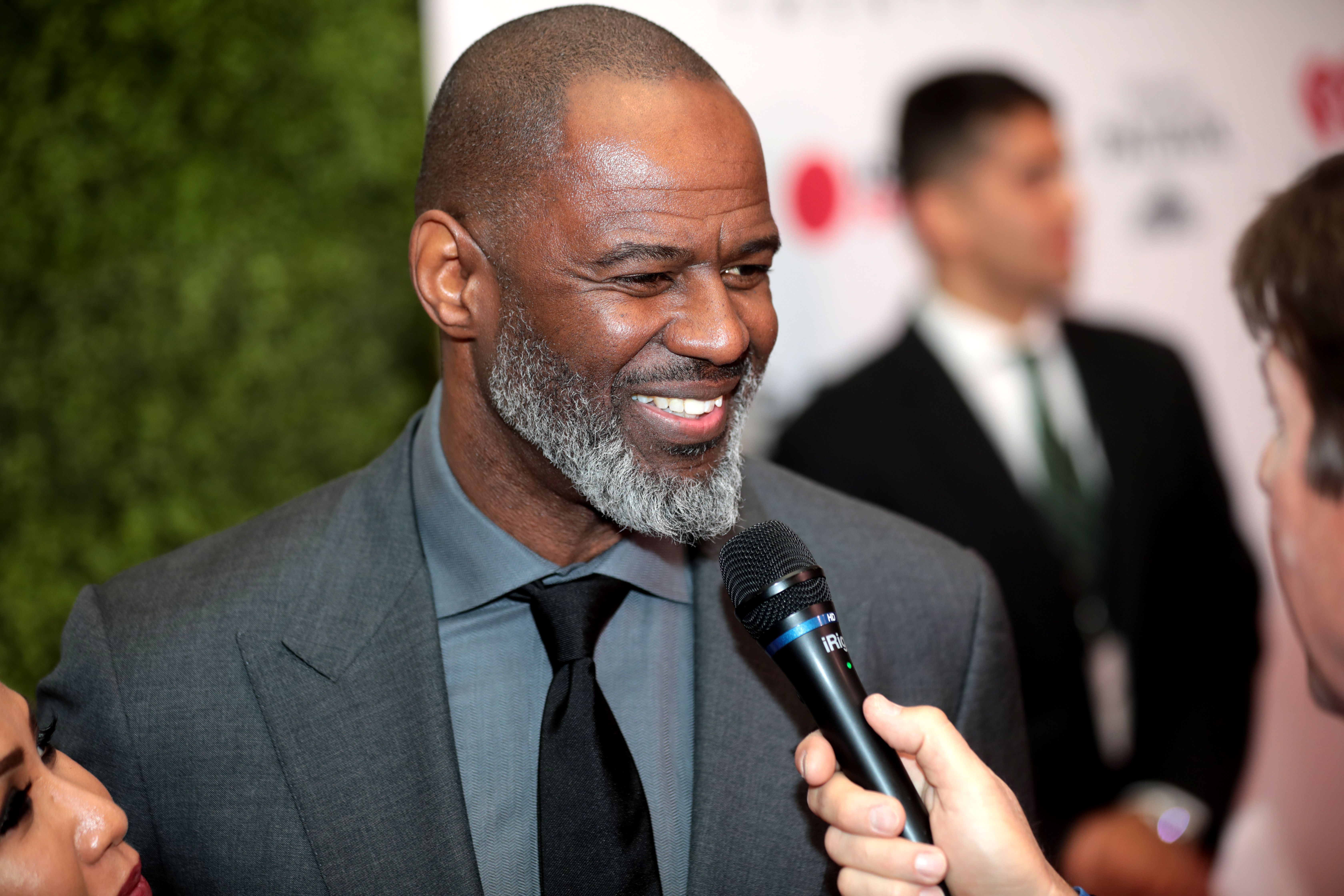The photograph captures an interview scene during what appears to be a formal event. In the center of the image, an elderly, clean-shaven black man with a white beard is highlighted. He is dressed in a grey suit, grey shirt, and black tie. Directly in front of him, a person partially visible on the right, is holding a black microphone with a distinct blue band, conducting the interview. 

The backdrop showcases a white banner adorned with various logos on the right side, and vibrant green plants on the left, adding a touch of nature to the setting. On the far right, there's a blurred figure in the background, wearing a black suit with a white shirt and a green tie. What appears to be a watch adorns his wrist, and he has short black hair and is clean-shaven. 

At the bottom left corner, a very partial view of a woman's face can be noticed, contributing to the perspective that this is a busy, attended event.